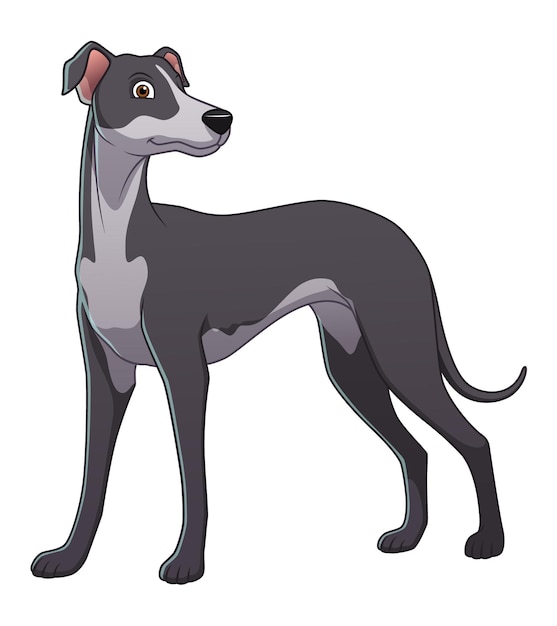The image is an illustration of a cartoon-like, tall, skinny dog resembling a Greyhound or Great Dane. The dog has a dark grey coat on its back, tail, and legs, transitioning to medium grey under its stomach and chest, finally blending into a light grey on its snout, neck, and the front of its chest. The chest features a unique light-grey marking that spans outward, almost resembling the shape of lungs or a guitar. The dog is depicted standing on all fours against a plain white background. 

The long, thin tail curls upwards at the end. The dog's large head is turned to the left, showcasing a black nose and a single, wide-open, surprised-looking eye with a dark iris surrounded by white. The face is primarily light grey, with a medium grey bottom jaw. Its floppy ears are grey on the outside and pink on the inside. The ears appear to stick up slightly before drooping at the ends. This detailed, computer-generated or drawn image effectively captures the whimsical and exaggerated characteristics of the dog.